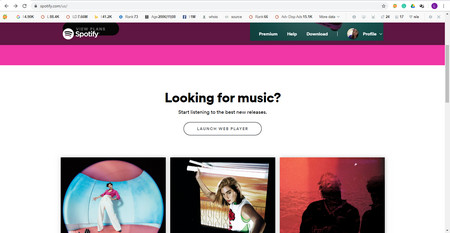This is a detailed screenshot of a Spotify webpage. At the center of the page, the text "Looking for music?" is prominently displayed, followed by a call-to-action that reads, "Start searching for" (the conclusion is blurry and unreadable), and a button labeled "Launch Web Player" underneath. Below this section, there are three distinct images: the first on the left shows a girl inside a ball; the middle image features a girl lifting what seems to be a window; and the third image on the right is a rap album cover with a red background and a black silhouette. At the top of the website, the Spotify logo is accompanied by a pink underline. There is a menu with options such as "Subscription," "Download," and "Profile," the last of which includes a small round profile picture. The webpage's overall design presents a white background with contrasting burgundy and pink accents. The browser window also shows several open, yet unreadable tabs, along with various icons on the top right. Additionally, there is a star for favorites and a bookmarked bar visible.